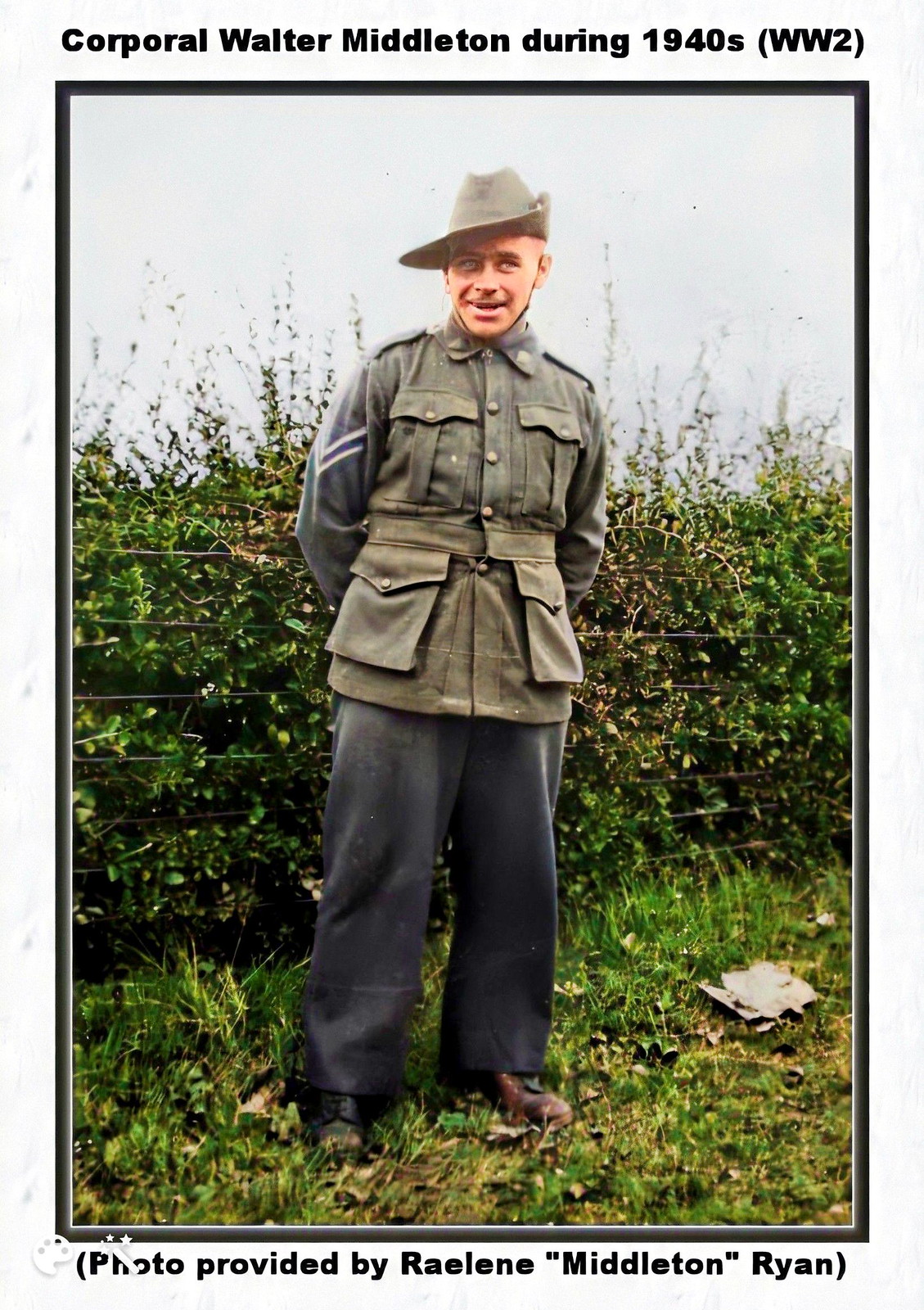This photograph features Corporal Walter Middleton during the 1940s World War II era. He is standing on grass in front of a wire fence with bushes behind it. Corporal Middleton is wearing a green-gray military-style jacket with two stripes on the arm, which is buttoned up, and black, rather baggy pants. He has on a brimmed hat with a strap that goes under his chin, one brim folded up and the other side sloped downward. He is smiling and looking slightly upward while facing the camera, with his hands clasped behind his back. The image has a black and white border, with black text above reading "Corporal Walter Middleton during 1940s, (WW2)" and below stating "photo provided by Raylene 'Middleton' Ryan."